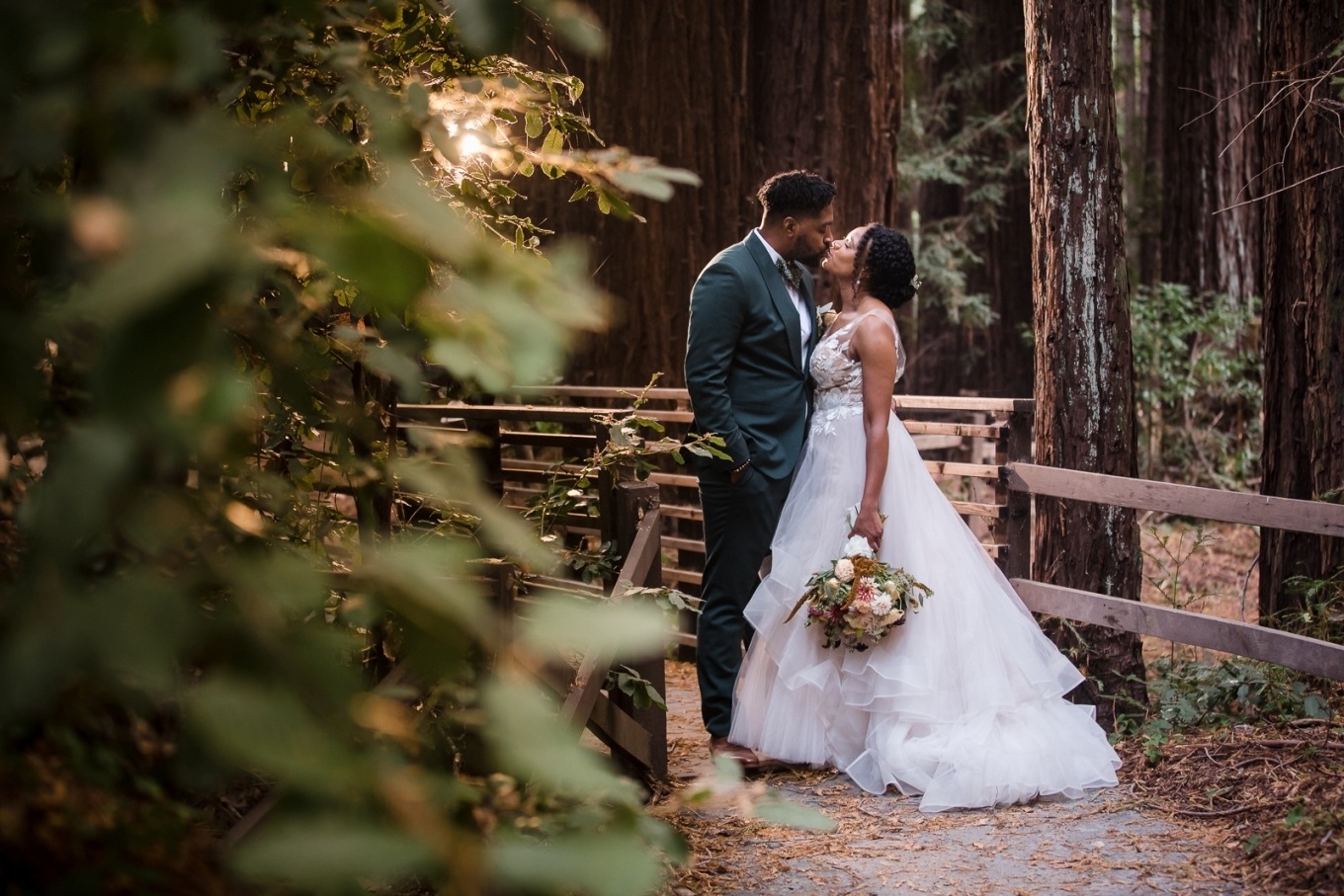In a serene forest setting, a man and a woman share a kiss on a concrete pathway, standing at the foot of a wooden bridge with fences on each side. The woman, situated on the right, wears a stunning, loose-fitting white wedding gown adorned with frills and lace at the bodice, which slightly presses into the man's stomach. Her elegant dress features tank top straps, and her brown hair is neatly pinned up. She holds a bouquet composed of white, tan, and light pink flowers in her left hand, which hangs by her side. The man, positioned on the left, is attired in a sophisticated black and white suit with a loose black tie and a dark green jacket. His right hand rests casually in his pocket, and his short black hair complements his outfit.

The background reveals a forest with tall, dark brown tree trunks, some bearing a hint of green-teal coloration. Leaves and branches frame the pathway, with many leaves blurred in the distance, contributing to the romantic and intimate ambiance. A yellow light glows softly from the top left, illuminating the scene and adding a warm, ethereal touch to the foliage and surroundings. The overall photograph captures a tender moment, possibly post-wedding, amidst the natural beauty of the forest, evoking a sense of timeless romance and tranquility.